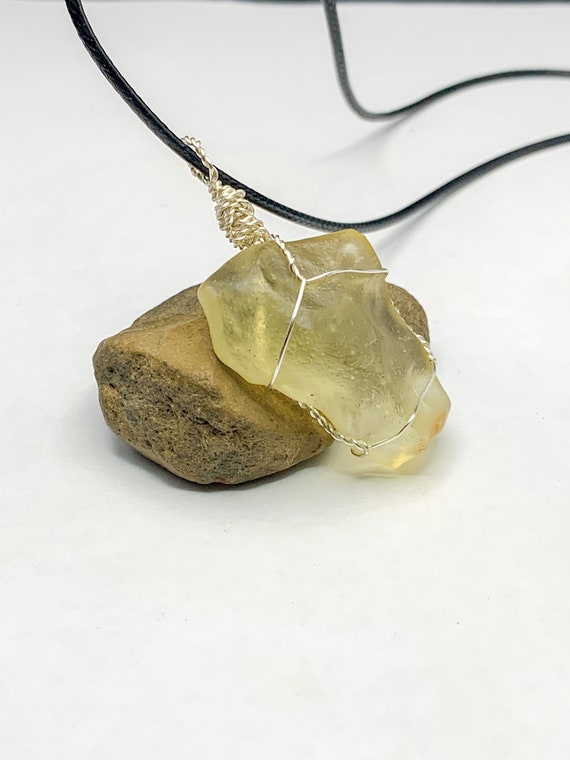In this image, a piece of jewelry is prominently displayed. The central focus is a pendant that appears to be a crystal, which is slightly opaque and exhibits a clear yellowish tint, hinting at its natural stone qualities. The pendant is intricately wrapped in silver wire, connecting it to a black leather cord that forms the necklace. This elegant piece is showcased by placing it on top of a smooth, brownish-grey rock with a textured, porous side visible on the lower left. The setting further enhances the pendant's detailed craftsmanship. The background is a light blue hue, providing a clean contrast and allowing the shadows of the objects to be subtly visible towards the bottom of the image.